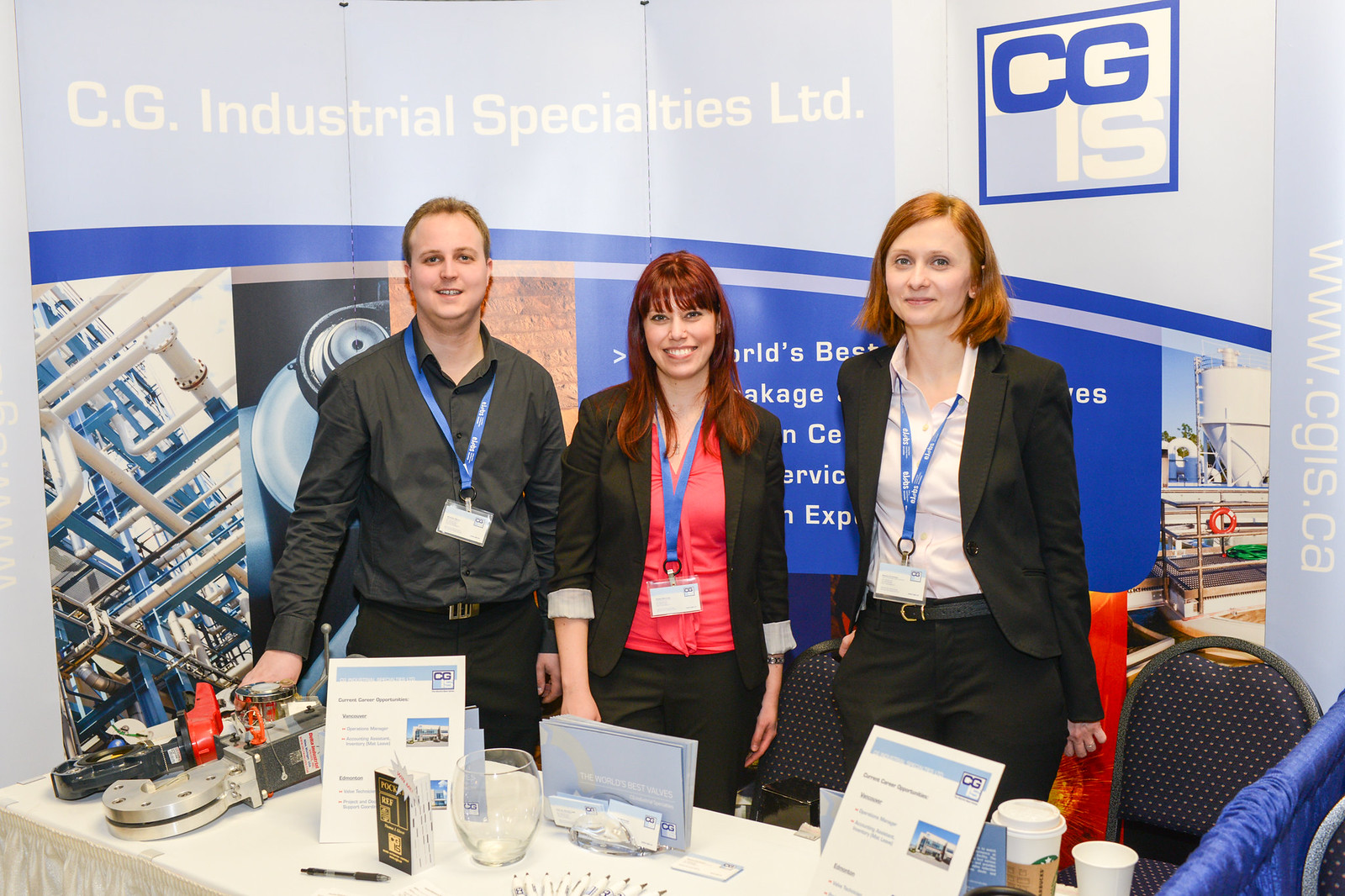The image depicts three young adults in their early 20s to mid-20s standing in front of a rectangular table covered with a white tablecloth, inside a room. The table is arranged with various items including brochures on stands, pens, buttons, note cards, business cards, a large open glass container, and some small metal tools. There are also drinking glasses and coffee cups scattered on it. All three individuals are wearing blue lanyards with laminated name tags around their necks.

On the left stands a man with short brown hair, smiling at the camera. He is dressed in a dark gray button-down shirt and black slacks. Next to him in the middle is a woman with long, reddish hair and bangs, also smiling. She is wearing a red button-down blouse with a black jacket over it and black slacks. The woman on the right has short, orangish-red shoulder-length hair, and dons a white button-down blouse with a black jacket and black slacks, smiling at the camera as well.

Behind them hangs a large banner in hues of gray and blue, with the text "CG Industrial Specialties Limited" displayed prominently in white letters across the top. To the right side of the banner is the CGIS logo encased in a blue border. The banner also features additional text and images of machinery, partially obscured by the standing individuals. Additionally, black and blue chairs with white dots are visible behind the table.